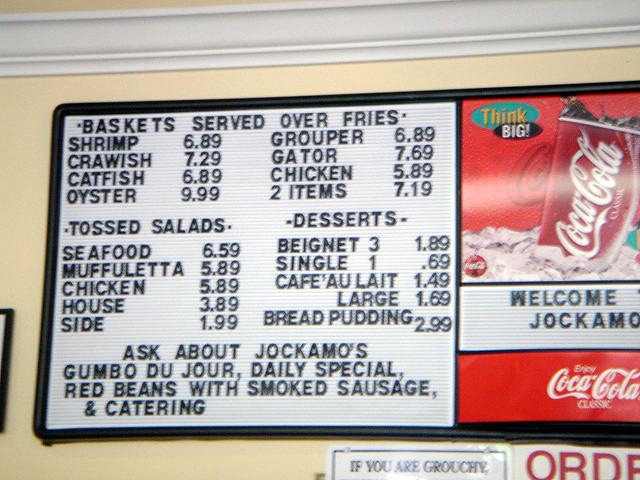The photograph captures a vivid scene of a Cajun-style eatery menu displayed on a wall. The menu features a classic, rearrangeable letterboard design in black and white, reminiscent of those often found in New York City pizza shops. It is mounted on a cream-colored wall, accented with white molding. The comprehensive menu lists a variety of offerings, including po'boys and baskets with shrimp, crawfish, catfish, oyster, grouper, gator, and chicken, with prices all comfortably under $10. There's also a selection of tossed salads such as seafood, muffuletta, chicken, house, and side salads, with prices ranging from $6.59 to $1.99. Desserts include beignets, café au lait, and large bread puddings, priced under $3.

Adjacent to the menu, a series of Coca-Cola advertisements add a splash of color. To the left, a large red Coca-Cola poster features a fountain cup of Coke with the words "Think Big" in a green and black bubble. Below that, a smaller interchangeable letterboard reads "Welcome Giacomo," with part of the word "to" visible below. Beneath this is a thinner Coca-Cola strip in red, displaying the classic "Enjoy Coca-Cola" slogan. Near the bottom of the photo, the letterboard menu begins to display the section starting with "Order," visible as "O-D" and part of an "E."

Further to the right, a tin sign with a partially visible black-bordered inscription begins with "If You Are Grouchy." The menu notably includes specials such as Giacomo's Gumbo Du Jour, daily red beans with smoked sausage, and catering options, emphasizing its authentic Cajun flair.